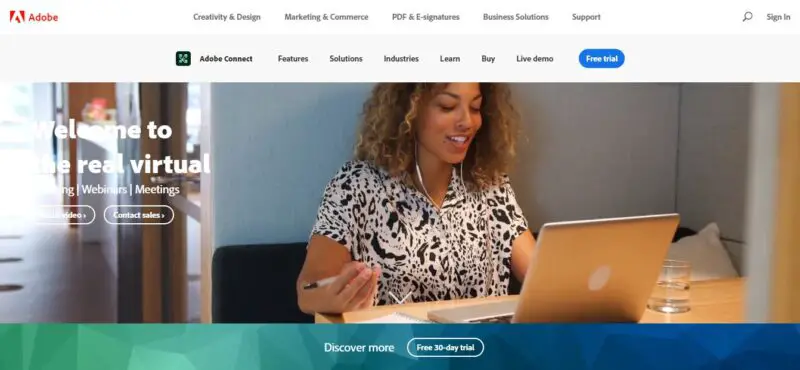The image displays a webpage showcasing an African American woman wearing a white floral shirt with black accents. She has short, curly hair and is adorned with a white headset. The woman is holding a white pen with a black tip and is seated in front of a silver Apple laptop, identifiable by the white circle logo on the back. She appears to be sitting on a blue bench with a white pillow to her right, against a backdrop of white walls, suggesting a home setting.

In the top left corner of the webpage, the Adobe logo is prominently featured—a red square with a white 'A' and the word 'Adobe' written in red next to it. Below this, in light gray text, are several clickable areas: 'Creativity and Design,' 'Marketing and Commerce,' 'PDF and e-signatures,' 'Business Solutions and Support,' among others.

Further down, there is a dark gray bezel followed by a dark blue symbol with a green X, next to which 'Adobe Connect' is highlighted in dark black. Additional black tabs are visible, including 'Features,' 'Solutions,' 'Industries,' 'Learn,' 'Buy,' and 'Live Demo.' There is also an olive, oval button with dark blue and white text that reads 'Free Trial.'

At the very bottom, a bezel transitions from teal and light blue to dark blue, ending in a very dark blue on the far right. In white text, it reads 'Discover More,' accompanied by an olive oval button bordered in white which states 'Free 30 Day Trial.'